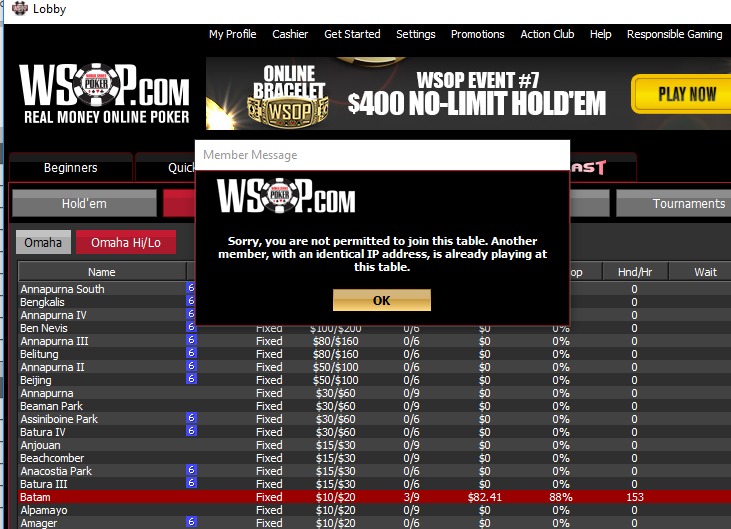A detailed screenshot image from the WSOP.com website is depicted. At the top, a white header features a semi-visible icon and the word "Lobby" in black text beside it. The page background transitions from black to gray, and in the upper left corner, the website name "WSOP.com" is displayed alongside its logo, with the 'O' creatively designed as a poker chip icon. Below this, the tagline "Real Money Online Poker" is prominently shown, followed by a navigation area listing options from left to right: Hold'em, Tournaments, Omaha, and Omaha High and Low. Superimposed on the page is a white and black pop-up message reading "Member Message" at the top and, against a black backdrop, the text "WSOP.com" followed by "Sorry, you are not permitted to join this table."